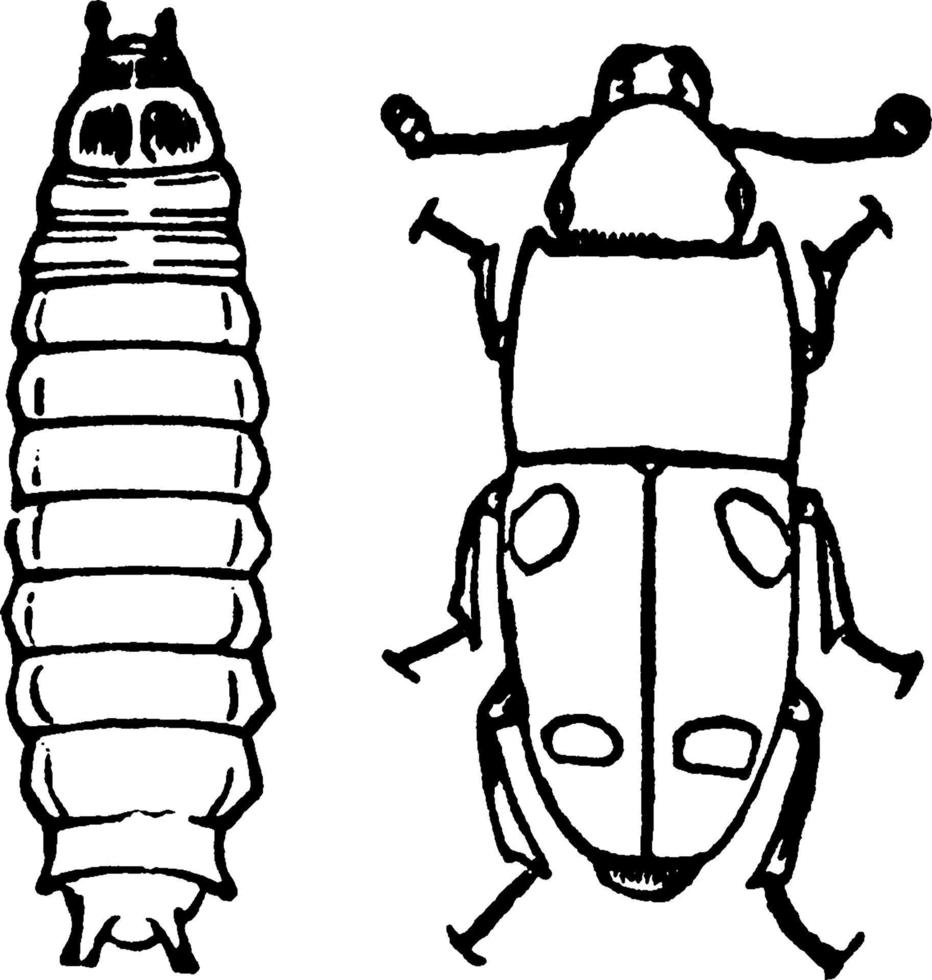This black and white drawing consists of two detailed ink illustrations. On the left is a long caterpillar-like insect with a segmented body comprising ten distinct sections and a rounded tail end featuring two protruding appendages. It has a head at the top with two short antennae and two black eyes, giving it a childlike yet thoughtful appearance. On the right side, there's a depiction of a beetle with a hard shell. The beetle's head has prominent pincers pointing forward and antennae on either side. It also features a head, thorax, and body where two wings sit, each marked with two spots. The insect has six legs, three on each side, drawn with visible detail. The entire illustration is rendered in black and white, suggesting the use of pen or marker and showing a high level of meticulousness likely from an adult artist.